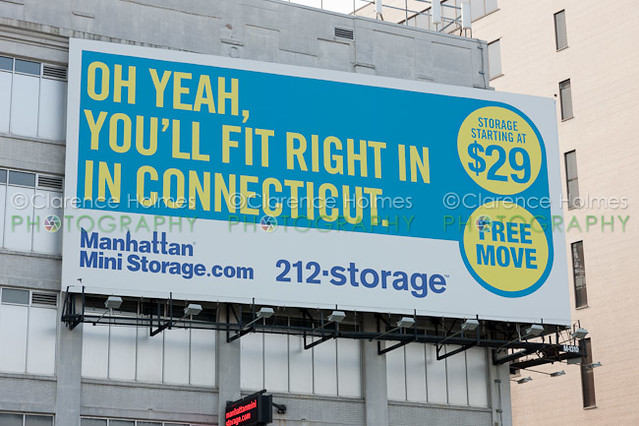This image showcases a vibrant billboard advertisement promoting storage solutions. Dominating the lower portion of the billboard is the website "manhattanministorage.com" and the phone number "212-STORAGE" written prominently in dark blue text. At the top, within a teal blue rectangle, the billboard features a cheeky blue text slogan: "Oh yeah, you'll fit right in in Connecticut." The right side of the ad highlights pricing information within two yellow circles; the first circle announces "Storage starting at $29," and the second adds "Free move," both in coordinating teal blue text. The entire image is slightly overlaid with a semi-transparent copyright watermark reading "Copyright Clarence Holmes" repeated three times, and the word "photography" in a lighter green hue, indicating the photographer's credit.